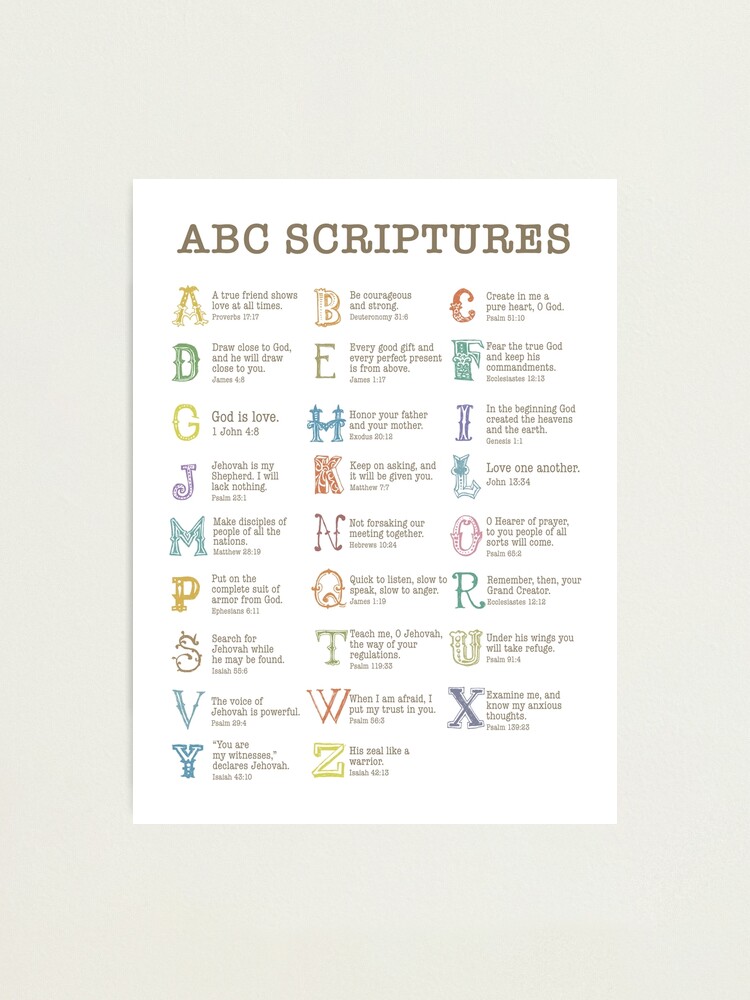The image presents a poster against a light off-white to yellowish background. The poster itself is white with the title "ABC Scriptures" displayed prominently in large, uppercase, brown text at the top. Below the title, the alphabet is arranged in three colorful columns featuring whimsical, pastel letters in hues of yellow, green, purple, red, and more. Each letter is artistically unique with intricate designs; for instance, the letter Q is adorned with little eyes and a nose.

Beside each letter, there is a corresponding scripture with a Bible verse, though the font is an old type style that makes it somewhat difficult to read. For example, next to the letter A, it reads, "A true friend who shows love at all times" with a reference to Proverbs 17:17. For B, it says, "Be courageous and strong," from Deuteronomy 31:6, and for C, the text reads “Create in me a pure heart, O God,” from Psalm 51:10. Another example includes, "God is love" next to the letter G, citing John 4:8. The letters and scriptures continue in this manner down to the letter Z. The background of the poster contrasts lightly against its surroundings, creating a soft and inviting appearance.